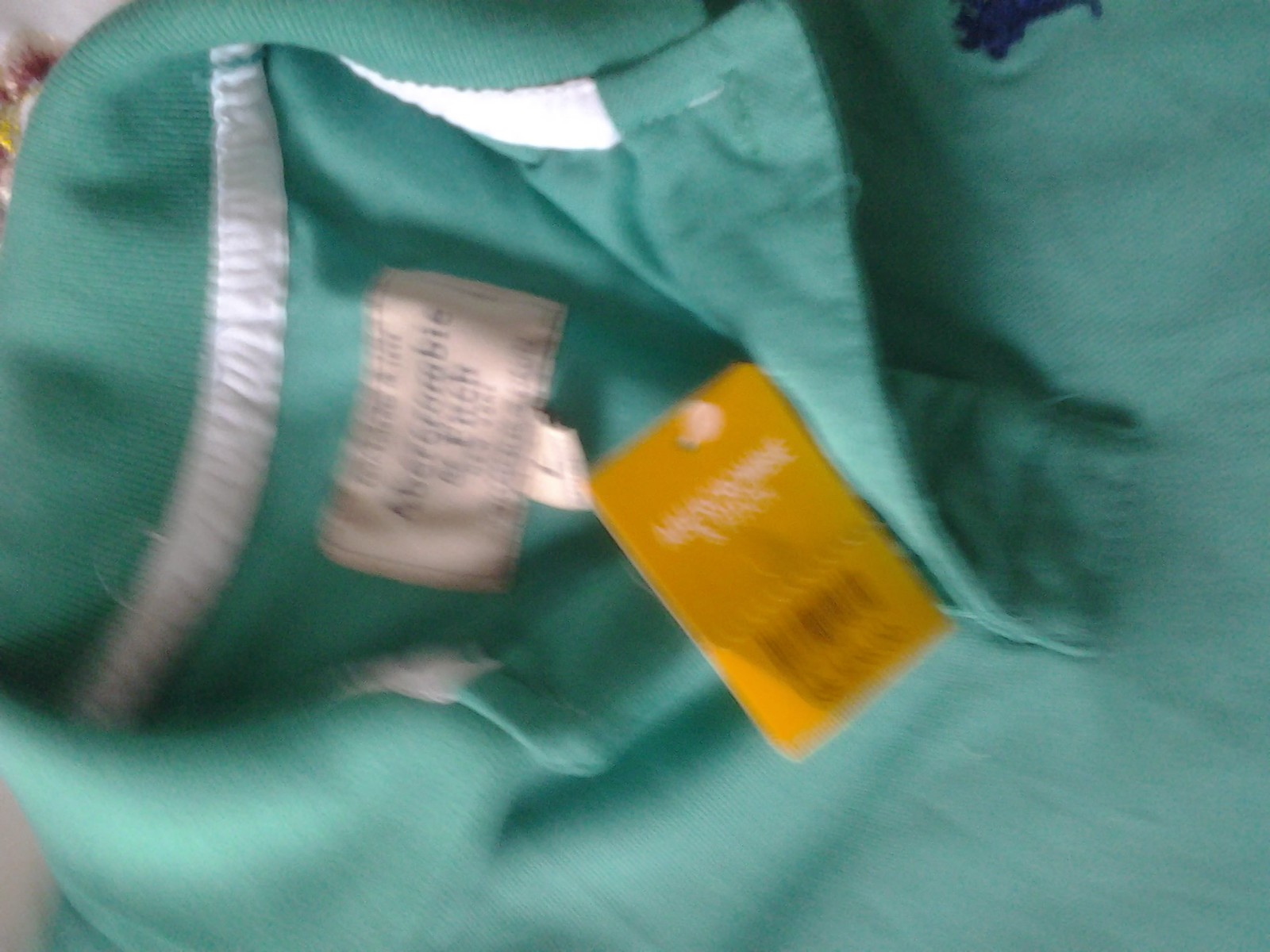The image features a very blurry photograph of a sea-green collared polo shirt, identified as Abercrombie & Fitch. Despite the blur, the Abercrombie & Fitch brand is discernible from the white fabric tag located at the nape of the collar. This tag is visible and clearly displays the brand name. Adding to this identification, a store tag with an orange barcode is visible beneath the brand tag, suggesting that the shirt may be new or has been recently purchased. Additionally, a small dark blue logo is positioned on the left breast of the shirt, further indicating the brand. The background of the image is indistinguishable, focusing solely on the polo shirt itself.